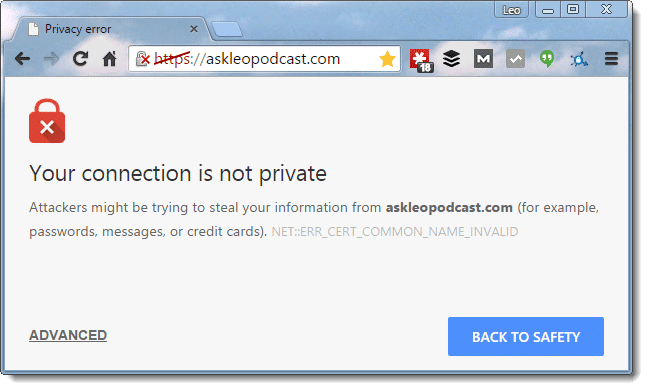This image captures a computer screen displaying a security warning pop-up from the website askleopodcast.com. The warning message features a red diagonal line cutting through the HTTPS in the address bar, which is accompanied by a red lock icon marked with an X. Dominating the pop-up is a bold message in large black letters stating, "Your connection is not private." Below this warning, a secondary message cautions, "Attackers might be trying to steal your information from askleopodcast.net. For example, passwords, messages, credit cards." 

The user is given two options: a smaller, all-caps "ADVANCED" link in black letters, and a larger, prominent blue button labeled "BACK TO SAFETY." The interface also includes various browser icons, such as a home button, reload button, and directional arrows for navigation. Additionally, there are multiple icons including a striking red square with a white snowflake-like design and the number "18" enclosed in a black box, an "M" in another black box, and various document icons. The upper portion of the screen displays an image of a sky with clouds, setting a stark contrast to the security alert below, with the browser tab itself labeled "Privacy error."